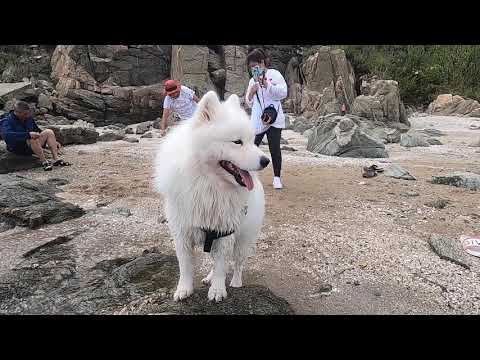In this outdoor daytime setting, the image captures a white Samoyed dog standing majestically on a rock, with its tongue playfully sticking out as it gazes off to the side. The dog is wearing a black harness that wraps around its neck and chest. Surrounding the dog are several people—two of whom are Asian women, each taking photos or recording videos of the scene. One woman wears a red hat and a white t-shirt, while the other dons a white sweatshirt complemented by a black purse slung around her neck and down to her hip. Additionally, a man in shorts and a blue jacket sits on a rock, looking downward, seemingly absorbed in something on the ground.

The backdrop features a ground predominantly made up of sand and sediment, interspersed with rocky gravel. Visible in the distance are various trees and bushes, enhancing the natural ambiance. The objects, including the dog and the people, are positioned near the center of the image, suggesting a focal point around the canine. The scene likely takes place in a public park or possibly a historical site, with colors ranging from tan, gray, brown, white, pink, red, blue, light blue, yellow, to green, adding vibrant details to the overall composition.